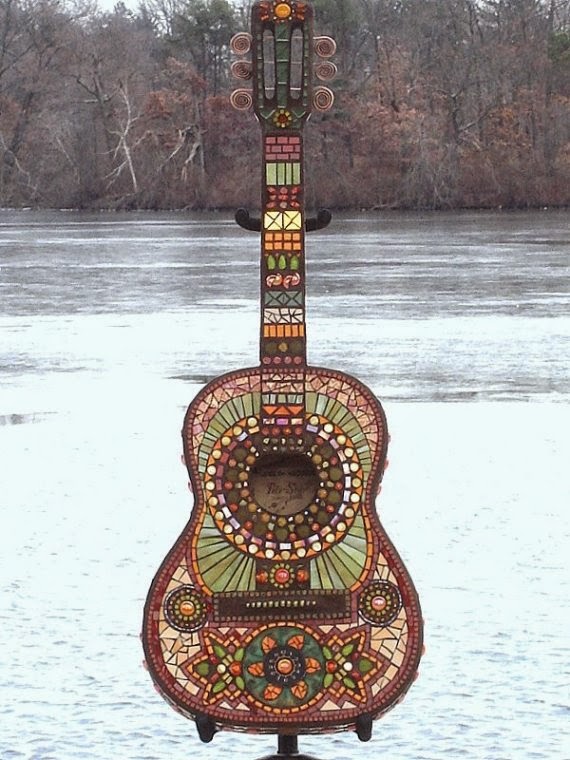This photograph, or photoshopped image, captures an intricately designed acoustic guitar standing upright on a post above a clear, flowing river or possibly a small lake. The setting appears to be during late autumn or early winter, with leafless trees and scraggly bushes lining the distant riverbank or lake shore under a clear blue sky. The water reflects the sunlight, adding a serene yet vibrant backdrop to the scene.

The guitar itself is an impressive work of art, transformed into a striking mosaic masterpiece. The entire instrument is adorned with a diverse array of colorful tiles, creating a complex and beautiful pattern that incorporates circles, squares, and sunburst designs. Each fret on the guitar’s fretboard features unique symbols or repeating tile designs, suggestive of Native American, Mexican, or South American influences. The decorative tiling extends to all parts of the guitar, even encircling the sound hole and various knobs, showcasing meticulous craftsmanship. This elaborate mosaic gives the guitar a timeless, almost sacred aura, making it appear as a permanent statue artistically placed by the water's edge.